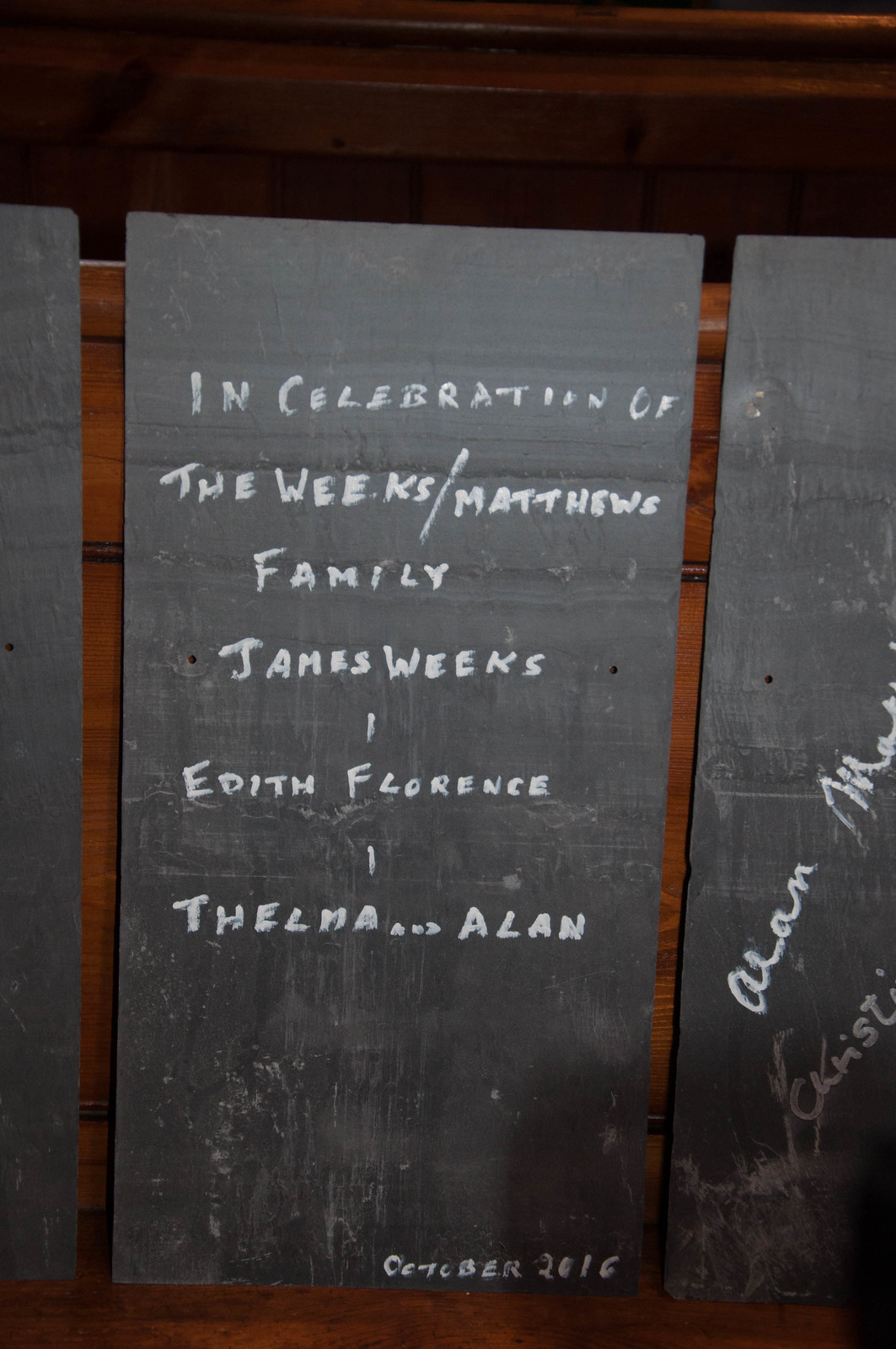This tall, rectangular photograph showcases a series of three chalkboards mounted against a dark brown, rich-colored, horizontal wooden plank surface. The central chalkboard is fully visible, framed by two others that are partially cut off by the edges of the image. The middle chalkboard features thick, white handwritten, all-capital letters that read: "In celebration of the Weeks-Matthews family, James Weeks, Edith Florence, Thelma Allen". In the bottom right corner, it is dated "October 2016". The chalkboard to the right also has white chalk writing visible, though it is partially obscured and appears to read names, possibly "Allen" and "Christy". This could be part of a commemorative piece, perhaps for a celebration of life or a family reunion, with some aspects resembling a memorial tribute where attendees may have added their signatures or messages.